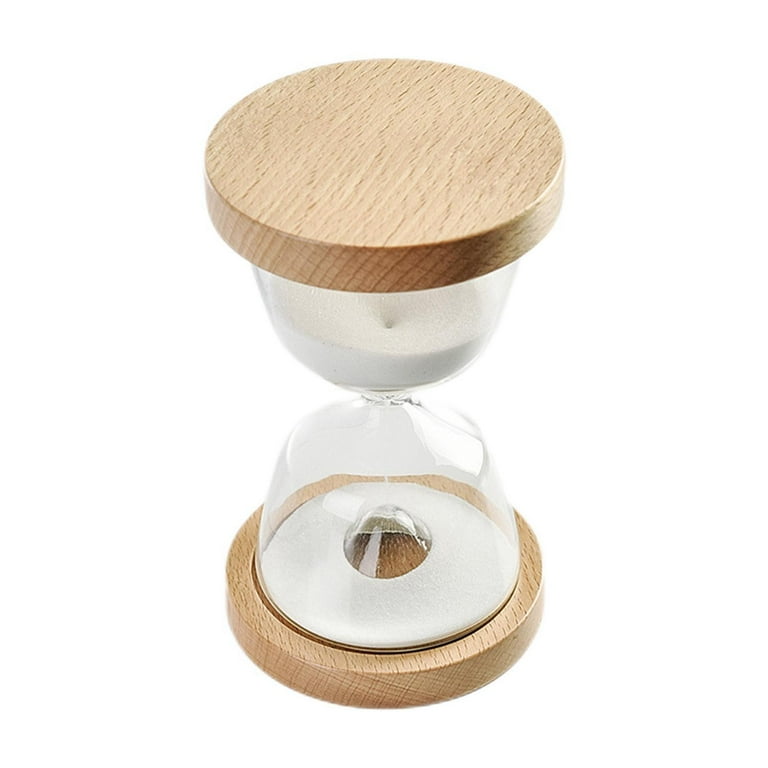The image depicts a small wooden hourglass with a white sand interior, set against a stark white background. The top and bottom sections of the hourglass are crafted in light brown wood, giving a warm contrast to the white sand. The hourglass is tilted slightly, offering a perspective that reveals the bottom part more prominently than the top. White sand is visibly trickling through the narrow neck from the upper to the lower bulb, forming tiny mounds that look like miniature mountains with snow cascading down. A considerable amount of sand remains in the top section, suggesting the hourglass has recently been flipped. This particular hourglass appears to be a smaller type, possibly used for measuring short intervals, such as timing eggs.